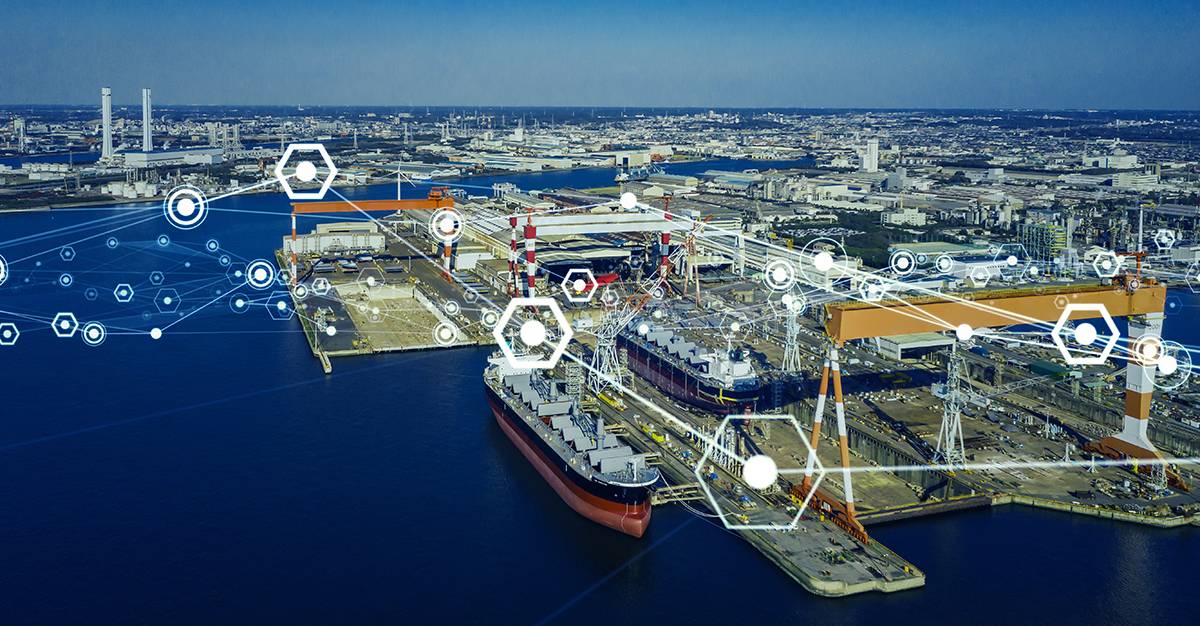The image depicts an industrial marina or port, characterized by a variety of large ships and vessels docked in the foreground. The deep, navy blue water occupies the lower and left sections, while the horizon is marked by the distant ocean and sky. Numerous multi-story white buildings extend along the horizon, with two tall smokestacks rising prominently on the left side of the image. The area is equipped with mechanical devices, cranes, platforms, and lifters, likely used for ship loading and manufacturing, suggesting that the port may handle cargo and the construction of large ships, perhaps including cruise ships.

Overlaying the image are several geometric shapes: octagons and hexagons with white circles inside them, connected by lines. These shapes and lines, which appear randomly placed, give the impression of digital or schematic elements possibly added via Photoshop. The presence of these figures, along with the surrounding industrial components, suggests engineers might use this image as part of visual area documentation, likely sourced from a specialized website. The juxtaposition of the city's infrastructure, mechanical elements, and deep blue water is harmonized in this detailed shot of a bustling port cityscape.